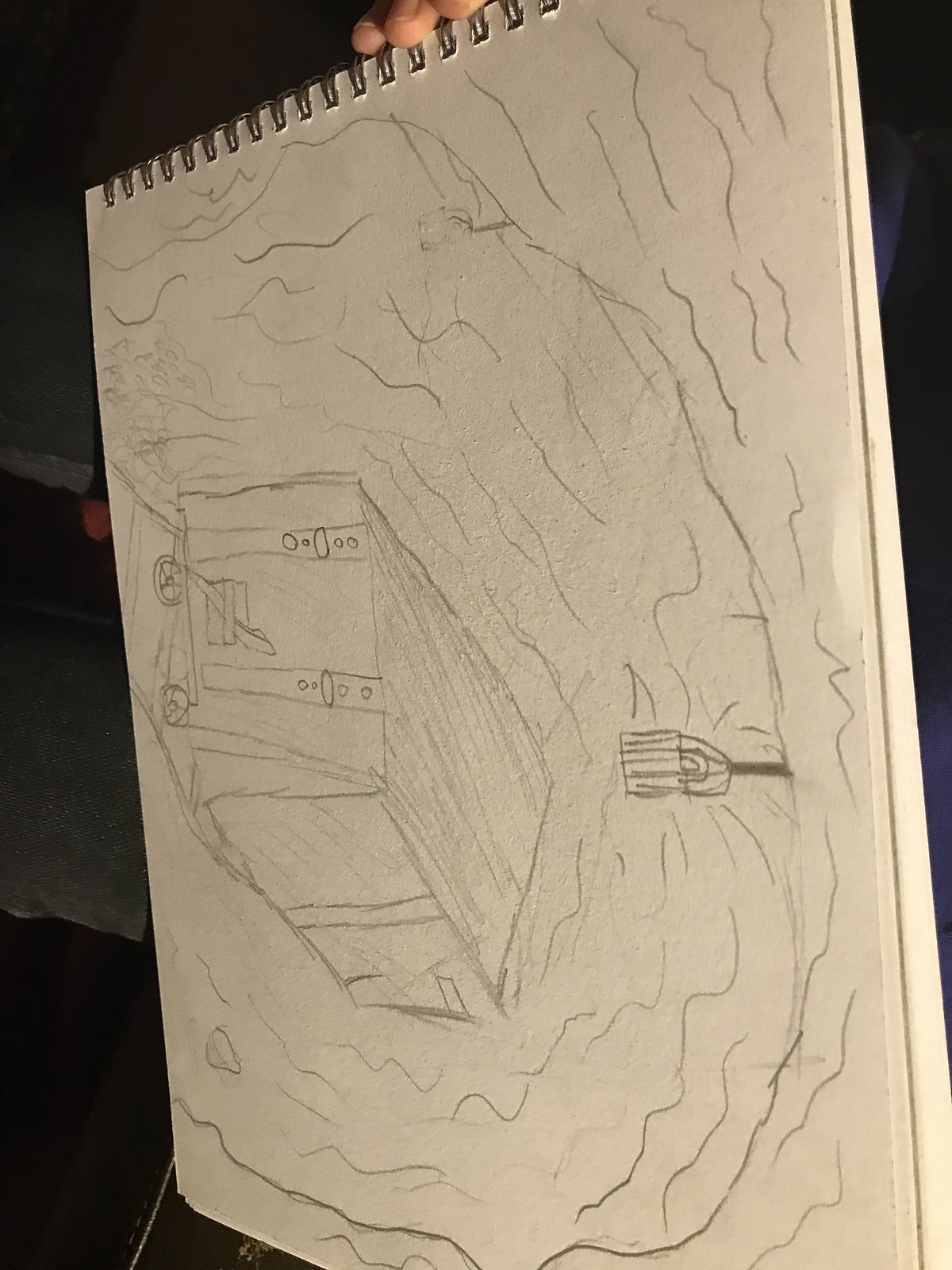This real-life photograph captures a close-up of a hand holding a spiral-bound sketch pad, prominently displaying a detailed pencil drawing. The sketch pad, held vertically, shows a landscape-oriented drawing, creating a visual juxtaposition that requires the viewer to tilt their head to fully appreciate the artwork. The visible fingertips grip the sketch pad from the top, ensuring the intricate details of the drawing are centered for the camera.

The artwork itself depicts a scene of a minecart emerging from a cave. The cave's textures and depths are intricately rendered with numerous lines, adding a sense of realism and dimension to the subterranean environment. From the cave's ceiling hangs a lantern, presumably illuminating the minecart's path along the faintly sketched tracks. The lantern’s inclusion suggests an adventurous or mysterious ambiance to the drawing.

The background of the photograph is cloaked in darkness, with indistinguishable shapes and shadows contributing to an overall atmosphere of mystery. This dark backdrop contrasts sharply with the white page of the sketch pad, drawing the viewer's focus entirely on the detailed cave drawing. No other elements are visible in the image, emphasizing the artwork and the hand that proudly holds it.